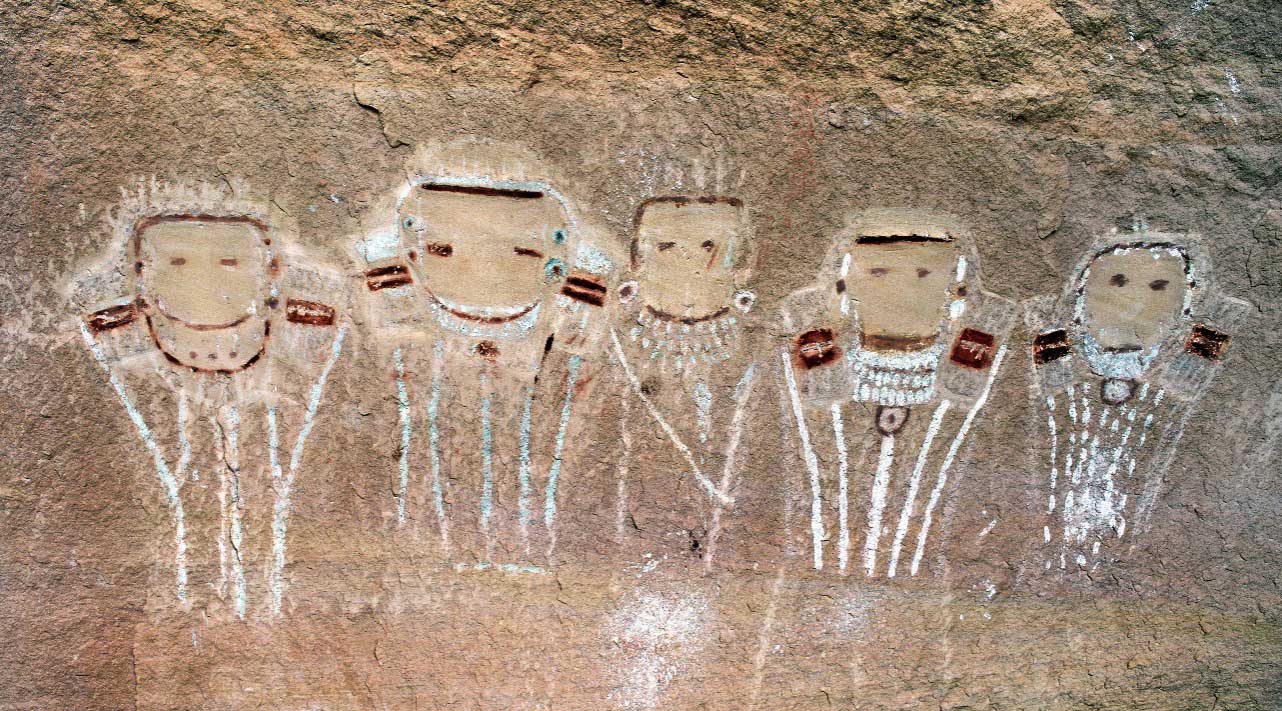The image showcases a light beige, rocky cave wall adorned with rudimentary paintings that seem to depict five human-like figures, reminiscent of ancient cave drawings. Each figure has a distinct form with wide shoulders and lines emanating from them, possibly representing clothing or adornments. The figures have simplistic faces with only eyes, depicted as small dots or lines. The artwork features various colors, including bits of turquoise, white, dark red, and brown, suggesting elements like jewelry or beading. The overall scene provides a vivid and detailed impression of primitive human art, capturing a glimpse of early human expression.